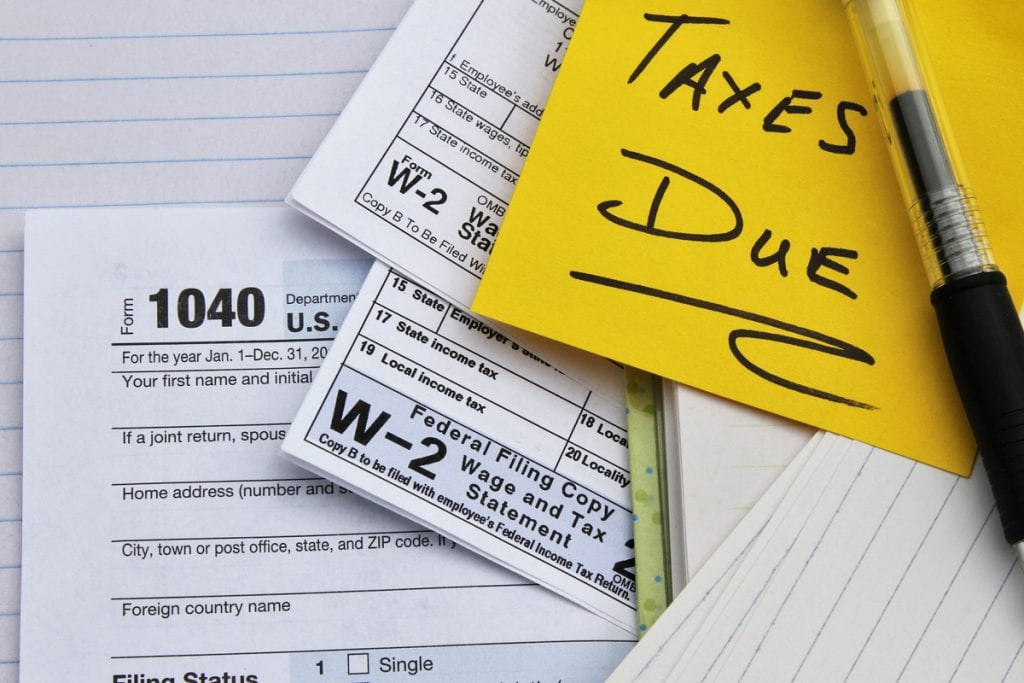In this close-up photograph, we see a detailed scene centered around tax paperwork, just in time for April 15th. Dominating the left side of the image, there is a partially visible IRS Form 1040, displayed atop a white piece of loose-leaf paper with blue lines. Overlaying the upper right corner of the 1040 form are two W-2 forms stacked together, clearly labeled as "Federal Filing Copy W-2 Wage and Tax Statement." Towards the right, a yellow sticky note prominently reads "taxes due," with the word "due" underlined in squiggly black ink. This note rests on the corner of the white paper and is paired with a black pen featuring a clear interior, which appears to be the implement used to write the reminder. In the lower right corner, there is a stack of criss-crossing index cards, rounding out the assortment of items in this well-organized, yet slightly cluttered, tax preparation scene.